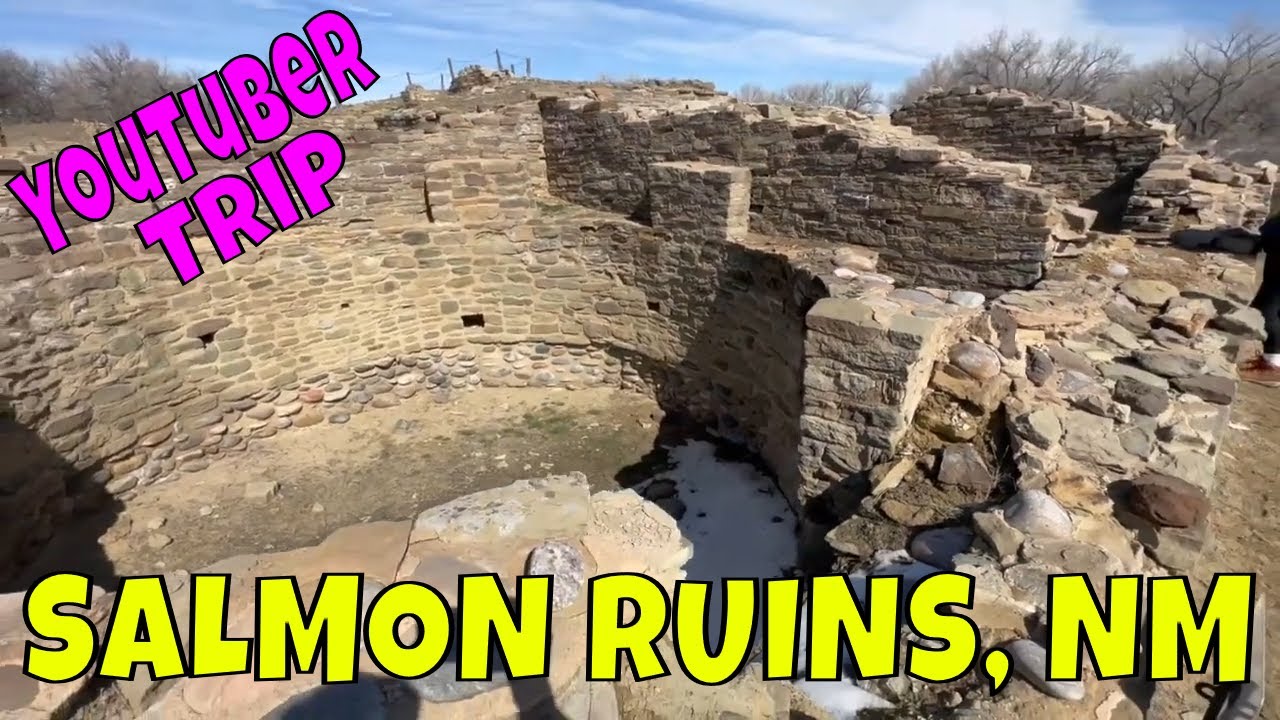This image appears to be a screen capture or perhaps a still from a video, highlighting the historical site known as "Salmon Ruins, NM" located in New Mexico. The top left corner of the image features the text "YouTuber Trip" in bright purple letters, while the bottom of the image displays "Salmon Ruins, NM" in bold, bright yellow all-caps letters. The background reveals a blue sky with scattered white clouds, with a prominent puffy cloud on the right side.

The focus of the image is the archaeological ruins, characterized by a large, circular structure made of brick and stone. The formation has multiple layers and appears somewhat haphazard, without a distinct shape reminiscent of modern architecture. The stone wall is composed of various shades of beige, tan, and gray, and is sealed with a substance typical of stone or brick buildings. The ruins, likely featuring some Native American historical elements, also include a central depression filled with water and rocks.

In the surrounding environment, there's a patch of dirt visible on the far right and a few trees without leaves scattered near the structure. Even though the stone formation looks old and somewhat dilapidated, it stands as an important and picturesque location, ideal for visitors interested in archaeology and history.